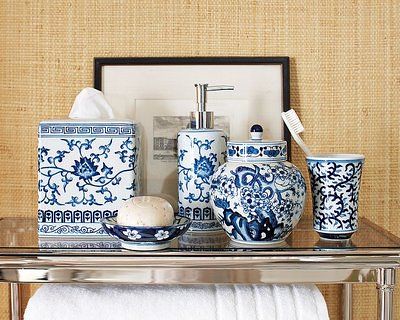The photograph captures a close-up view of a silver table positioned against a yellowish-colored wall. The top, sides, and three legs of the table are visible. Beneath the table, a white towel is draped over a chair. On the table, five bathroom accessories, all featuring blue and white designs, are neatly arranged. 

At the far left, there is a tissue box with a tissue slightly protruding. In front of the tissue box sits a soap dish holding a tan-colored, circular bar of soap. In the center of the table, there is a soap dispenser topped with a silver pump. To the right of the dispenser is a lidded container resembling a vase. Finally, at the far right, there is a toothbrush holder containing a single white toothbrush. 

Behind these items, a white picture frame with a brown outline stands, partially obscuring its contents. The overall composition creates a tidy and aesthetically pleasing arrangement of bathroom essentials against the backdrop of the subtly colored wall.